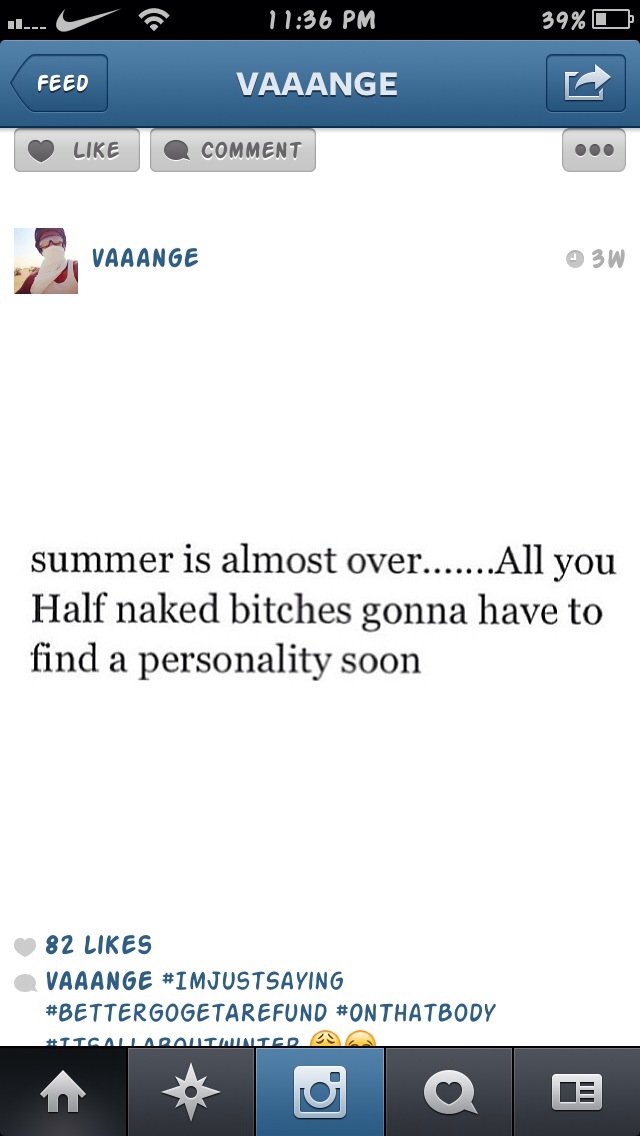This image is a vertical screenshot from a smartphone app. The top of the screen features a standard black bar with a Wi-Fi icon, the Nike swoosh, the time "11:36 PM," and a battery icon indicating 39% charge. Below this black bar is a blue section with "Vange" (spelled V-A-N-G-E) centered in light blue text. On the left side of this blue bar is a "Feed" button and on the right side, a forward arrow icon.

Beneath the blue bar, there are icons for liking, commenting, and an ellipsis (options menu). Following these buttons is an avatar showing a cartoony face, and text next to it reads "Vange" with a timestamp indicating "3W" (three weeks ago). The main content of the post states: "Summer is almost over... All you half-naked bitches gonna have to find a personality soon," written in left-aligned black text. Below this, the post has accrued 82 likes, indicated by a heart symbol.

The text at the bottom reads "Vange," followed by several hashtags: "#I'm just saying," "#better go get a refund," and "#on that body." Additionally, there are standard navigation icons at the bottom for home, Instagram, liking, and more, making the interface easily recognizable as a social media platform.